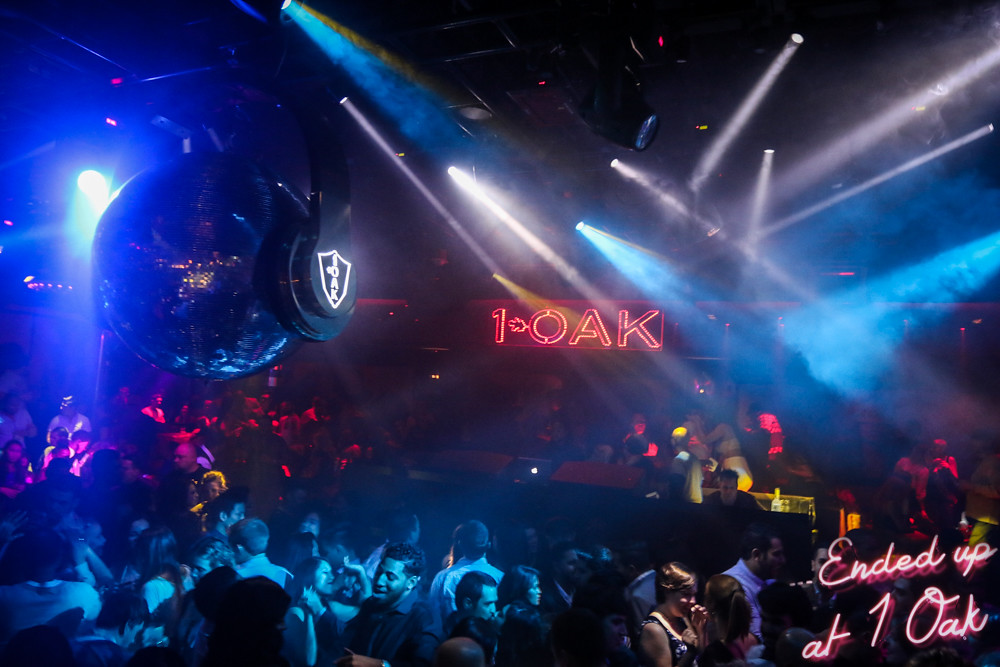The rectangular photograph captures a vibrant indoor scene inside a bustling dance club. The high-ceiling venue is illuminated with a plethora of lights, predominantly white, with accents of blue, yellow, and red, creating an energetic atmosphere akin to a typical night club. A notable illuminated sign in the center reads "1 OAK," framed with a red fluorescent oak leaf, representing the club's name. The bottom right corner of the image features an overlay in handwritten fluorescent text, stating "Ended up at One Oak," suggesting a social media post.

To the left of the sign hangs a disco ball adorned with over-ear headphones, adding a unique touch to the decor. Beneath the lights and sign is a dense crowd of people, dancing, chatting, and enjoying themselves in what appears to be a lively and packed environment. There’s a section that looks like it could either be a DJ booth or a bar, casting a yellow glow despite the overall dimness of the room, contributing to the club’s vibrant yet moody ambiance. The scene is further colored by shafts of blue and white light streaming from overhead, and the air has a slightly smoky quality, enhancing the overall nightclub experience.